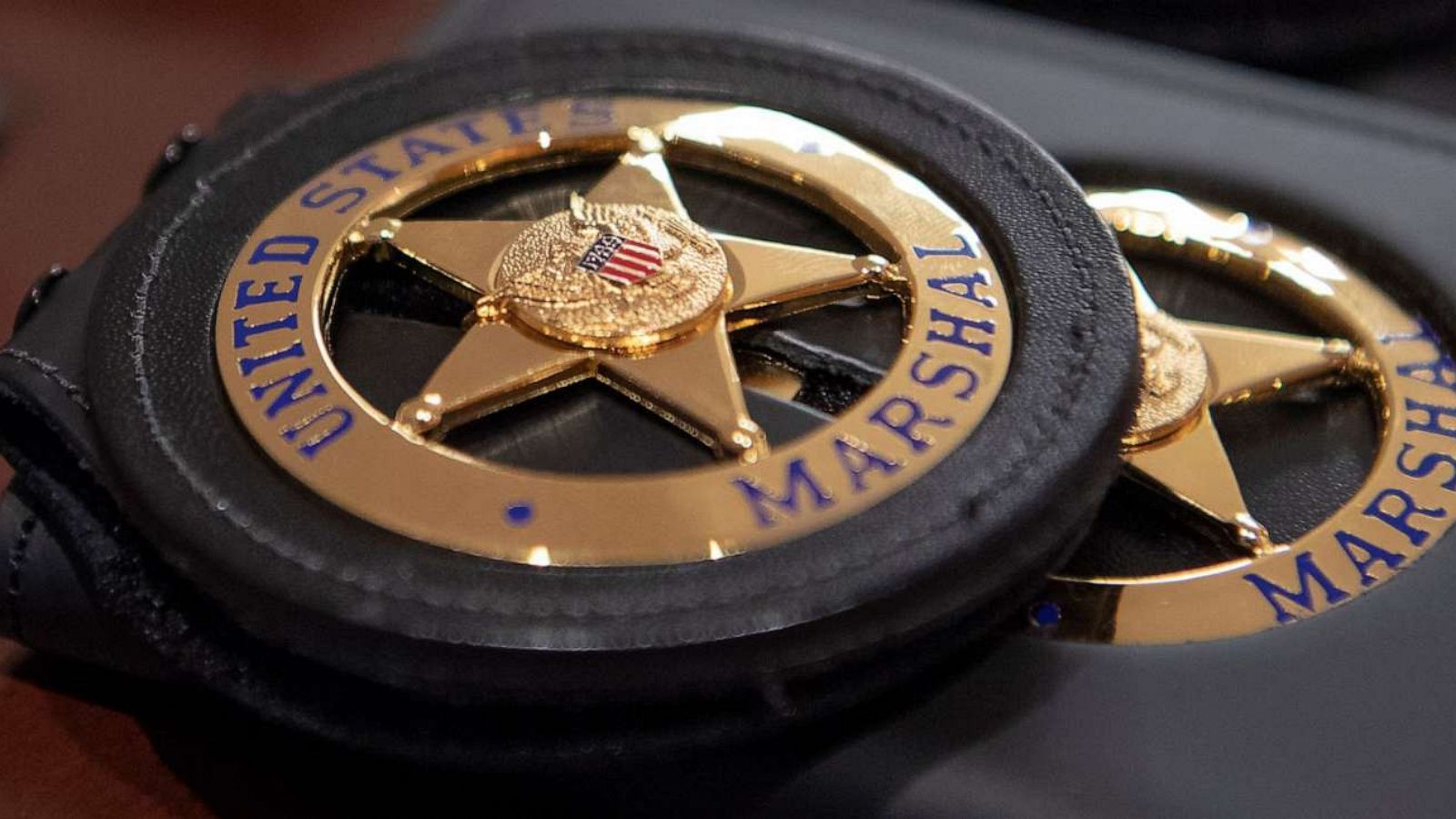The photograph, in landscape orientation, features a close-up of two United States Marshal badges arranged on a table. The upper badge is encased in a round black leather case with neat stitching, showcasing a golden or brass star at its center, bearing a textured, raised circle which encloses an American flag shield. The top of the badge reads "United States" in royal blue, while "Marshal" is inscribed at the bottom, also in royal blue. This badge partially obscures another below it, which is similar in design. The lower badge is set into a black rectangular leather wallet-like holder with a visible cutout. Despite being partially hidden, this badge also shows the same distinctive royal blue lettering and star design. The background is dark brown to black, contributing to a realistic yet somewhat stylized and possibly artificially generated feel to the lighting of the photograph.